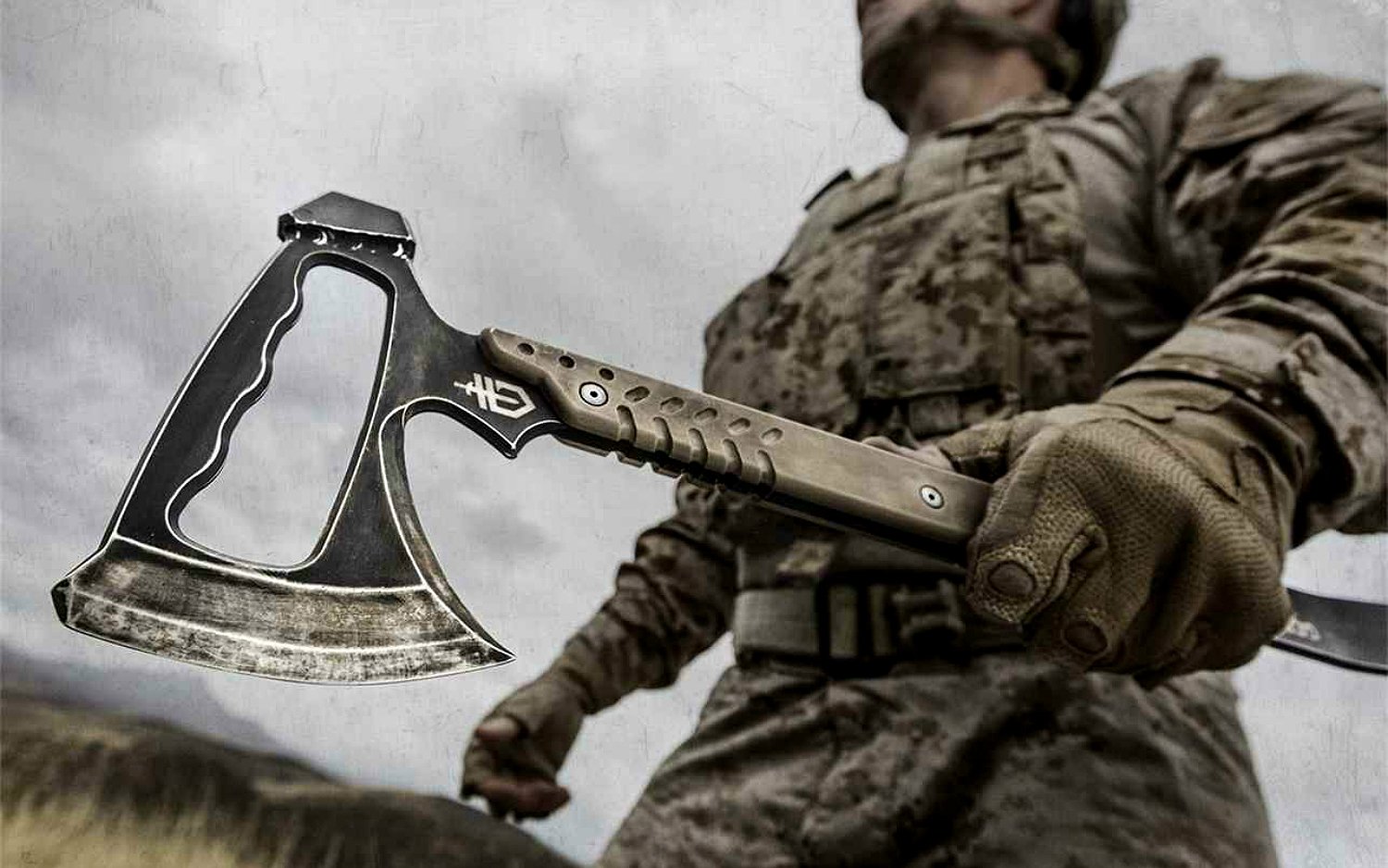In this detailed and gritty image, we see a soldier, dressed in army camouflage fatigues, positioned predominantly on the right side of the frame. This photo captures him from his hip up to his neck, emphasizing his rugged appearance in the wilderness. His left hand firmly grips a military-issue axe, featuring a beige handle and a distinctive black blade with a hole near its top. The axe's blade, appearing rusty and worn, points downward, dominating the central part of the image. The soldier's other hand, clad in a tan utility glove, hangs to his side. His helmeted head is turned slightly to the left, looking into the distance. The backdrop features a vast, grayish-white sky with dark, brown land visible at the lower left, enhancing the sense of remote wilderness. The overall color palette includes green, black, gray, yellow, beige, and brown, contributing to the gritty feel of the scene.